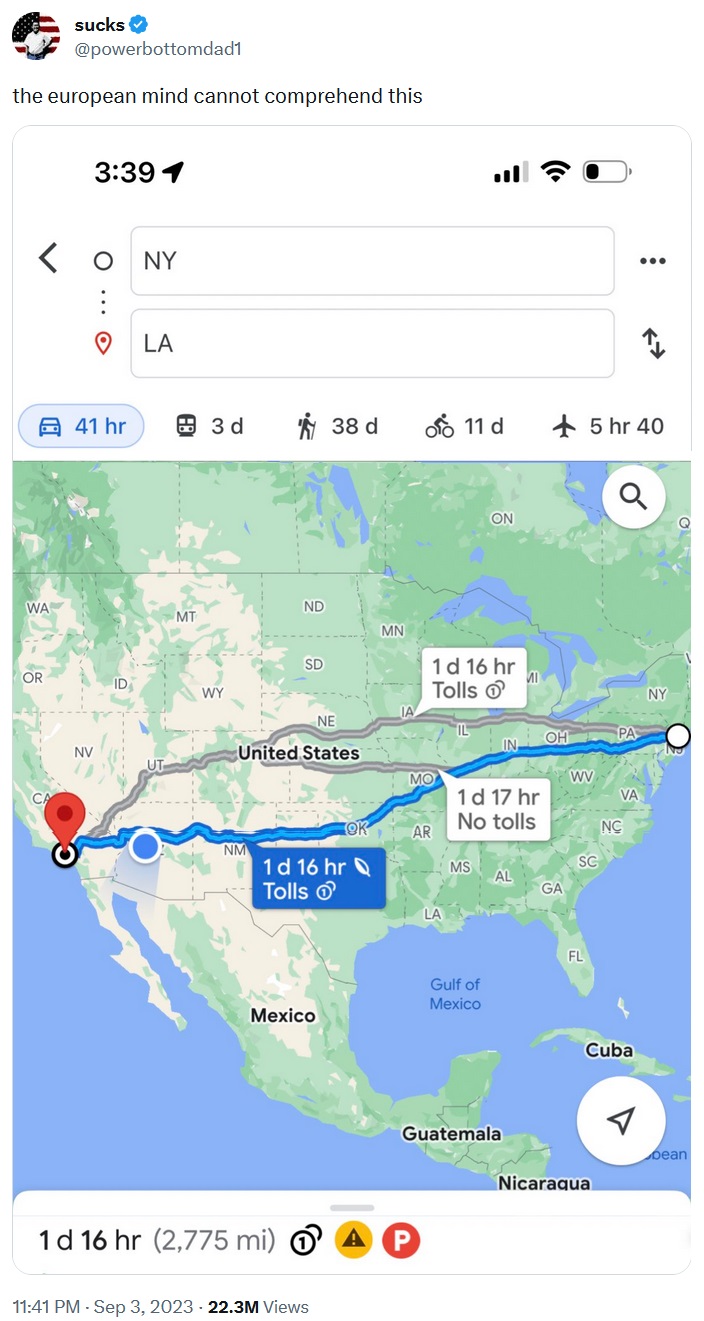Screenshot of a tweet by user "sucks" (@powerbottomdad1), verified with a blue checkmark. The profile picture features a man standing against an American flag backdrop. The tweet reads: "The European mind cannot comprehend this." Below the text, there is an image showing directions from New York to Los Angeles, accompanied by two white boxes with additional details. Beneath these boxes, five icons represent different travel methods and their estimated times: by car (41 hours), walking (3 days), biking (38 days), flying (11 days), and another mode seemingly indicating a plane (5 hours 40 minutes). A map displaying the route from New York to L.A. is included, with a red pin marking Los Angeles.

(Note: The "11 days plane" might be a mistake in the provided description since plane travel is listed again with a different duration of "5 hours 40 minutes.")